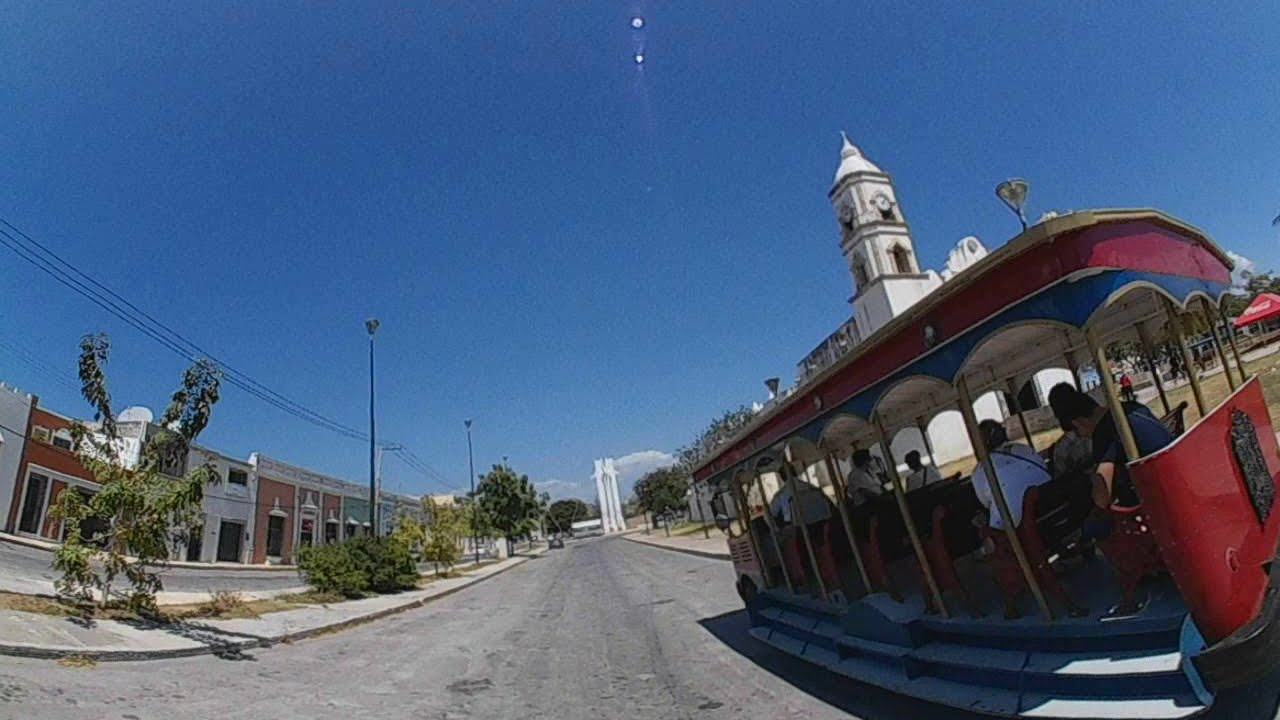The image captures a vibrant red trolley with a maroon body and red roof, navigating down a gray, paved street marked with oil stains and tire marks. The trolley features a blue canopy lining at the bottom and is supported by brown poles. Inside, a number of people are seated, including one person in a white shirt with a black line across the chest, resembling a purse strap, and another person in a blue shirt leaning forward in the back.

The street scene is shot with a distorted lens, creating a sense of the sides coming together. The right side of the street is partially obscured by the trolley, but a white, ornate building, possibly a church, with a pointed steeple and a clock is visible. There's also what appears to be a green park area and a red-topped gazebo in the background. On the left side, a series of one-story buildings in red, white, and blue, line the street amidst light poles, power lines, and trees. Decorative plants grow in a central berm where more lights are installed. 

In the far distance, a white tower rises at the end of the street against a dark blue sky with a few specks of white clouds.